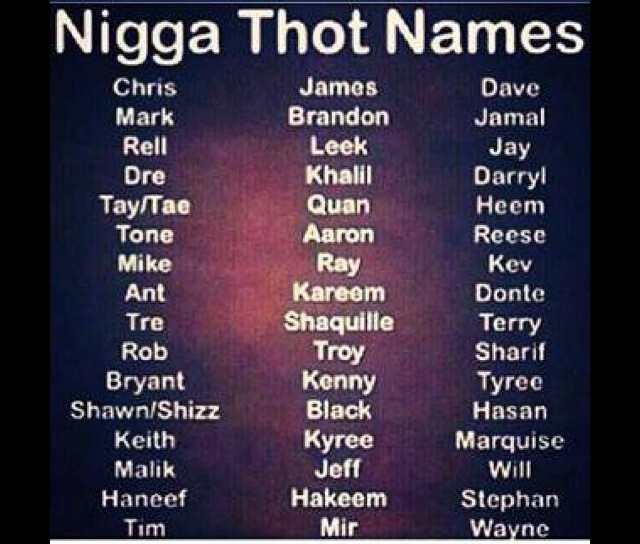This image appears to be a low-resolution, pixelated screenshot, likely taken from a YouTube video or similar source. The image is framed by black bars on either side, giving it an old-fashioned feel. The background shows a gradient that transitions from dark pinkish colors to dark purple. Centered prominently is a bold headline in white text reading "Nigga Thought Names" (N-I-G-G-A, T-H-O-T), situated above three columns of men's names. These names are listed in white text and are not organized alphabetically. The columns start with "Chris" in the first column, "James" in the second column, and "Dave" in the third column, continuing down with various common names until the last names in each column: "Tim," "Mir," and "Wayne." The overall design of the image combines photographic elements with clear typography, creating a visually structured list amidst the colorful gradient background.